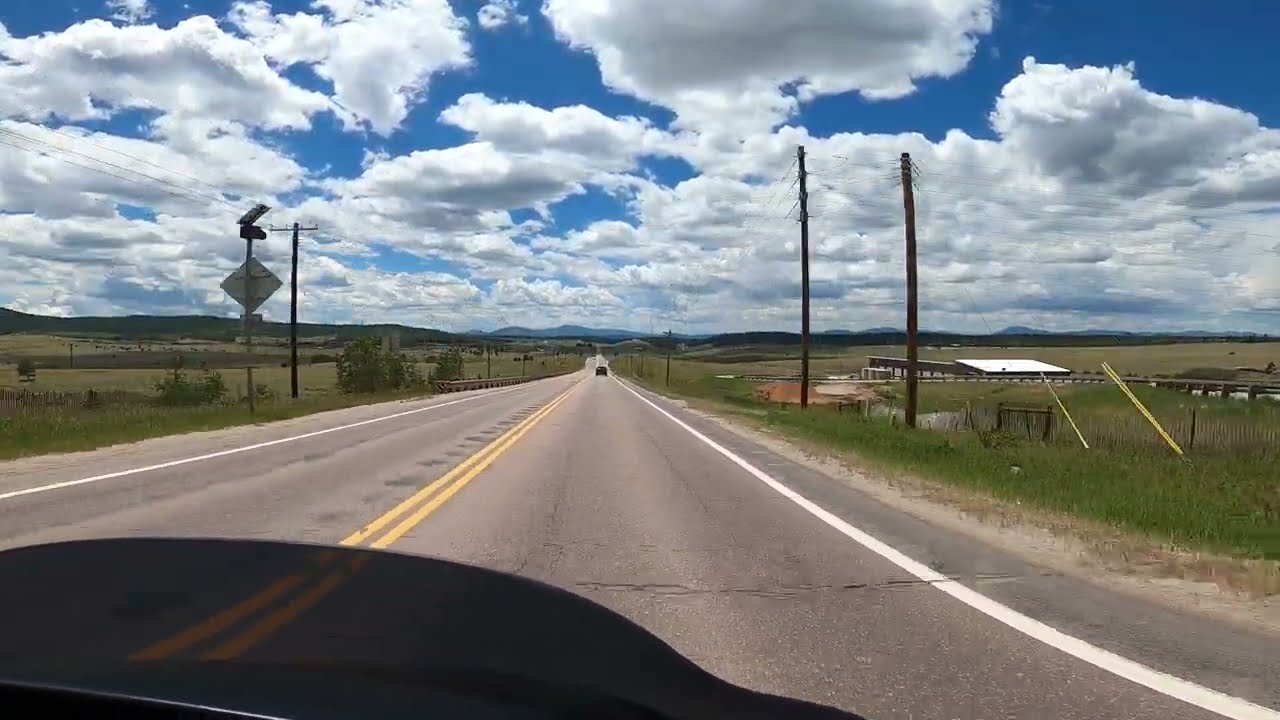A daytime point of view shot from a dash cam captures a drive down a cracked light gray asphalt road that stretches into the horizon. The road features solid white lines along its edges and a double yellow line in the center, dividing the lanes for oncoming traffic. Vast, flat green prairies spread out on both sides of the road. To the right, a fence encloses multiple single-story, flat-roofed buildings, possibly stables or barns, with telephone poles and wires running parallel to the road. A dark-colored car is visible further up ahead. On the left, green grass dominates the landscape, interrupted only by a diamond-shaped road sign facing the opposite direction. The top half of the image is filled with a big blue sky and large, fluffy white clouds, suggesting a sunny day. Toward the distant horizon, the silhouette of mountains or hills can be seen, enhancing the scenic rural atmosphere.